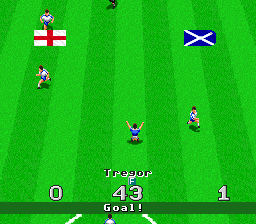A nostalgic screenshot of an 8-bit style video game captures an intense soccer match on a retro-styled field. The textured green field features symmetrical lighter and darker green stripes, adding a unique charm. In the heat of the moment, a triumphant player in the center, dressed in blue, raises their arms in celebration, having just scored a goal. The scoreboard at the bottom reads "Traeger 43 goal 0-1," marking the lead. The game appears to be between two teams, represented by their country flags: one with a white background and a red cross, and the other a blue rectangle with a white X. Additional players, adorned in either blue or white and red kits, can be seen in action. A player in white and red runs towards the right corner, another dashes to the left, while a third player near the upper side and close to the flag is sprinting to the right. The screenshot encapsulates the dynamic and vibrant atmosphere of classic video game soccer.